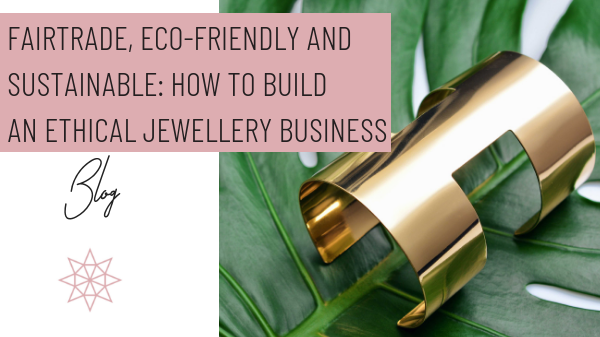The image is a detailed blog tagline for a jewelry website, featuring a vibrant design and promoting ethical business practices. The upper left corner showcases a pink box with black text that reads "fair trade, eco-friendly and sustainable: how to build an ethical jewelry business." The word "blog" is written beneath in a stylized cursive font, accompanied by a sun symbol composed entirely of pink triangles. The background is mostly blank white space. However, a notable feature on the right side is an image of a green, matte, possibly plastic leaf, which has a piece of shiny, cylindrical gold jewelry on top. This jewelry appears to be a bangle, perhaps resembling a bracelet that could be worn around the wrist or forearm.